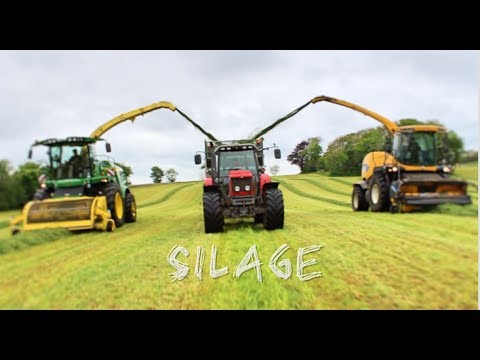The image features a detailed color photograph of three pieces of farm equipment situated in a grassy field under a cloudy, gray sky. The top and bottom of the photograph are bordered by horizontal black bars. Prominently displayed in white letters at the bottom of the image is the word "Silage," spelled out as S-I-L-A-G-E. 

The machinery is depicted as follows: On the left is a green and yellow harvester with a large yellow wheel in front and an operator visible on top. In the center, there is a red tractor with a bucket attachment and enclosed cab, flanked by the other two machines. On the right, a yellow and black harvester with an enclosed cab and visible operator matches the style of the one on the left. Both harvesters have long yellow arms extending toward the central red tractor, appearing to pour the harvested crop into its bucket. The field is dotted with rows of freshly cut yellowish-green grass, adding texture and context to the scene. In the background, a line of trees stands beneath a sky with grayish-white clouds, suggesting a break in the overcast conditions.